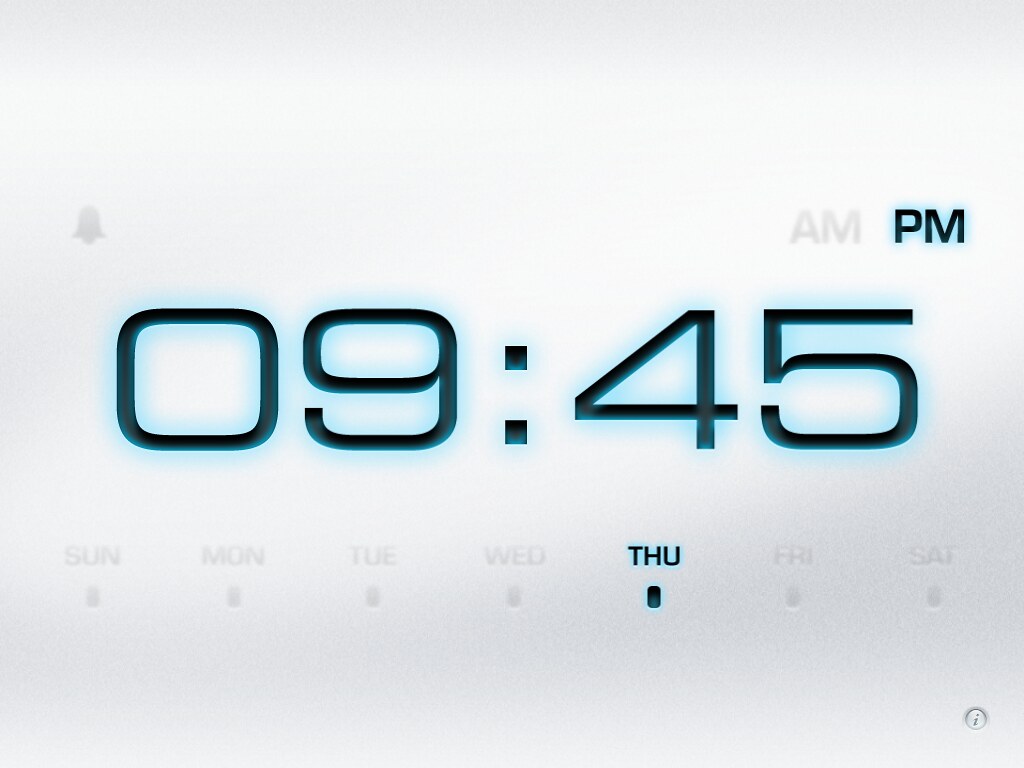This image depicts a digital alarm clock display, likely from a phone or computer interface, set against an all-white background. At the top, there is a thin gray line extending across the width of the display, with a small gray bell icon situated near the top left. Moving rightward, there is a gray 'AM' marker, alongside a bolded black 'PM' marker indicating that the selected time is in the evening. Centrally, the time is displayed in bold black as 09:45, bordered with a subtle light blue glow. Below the time, the days of the week are listed: SUN, MON, TUE, WED, THU, FRI, and SAT, each with a dot underneath. The 'THU' (Thursday) section is highlighted in black with its dot filled in, signifying that the current day is Thursday. The numbers and active elements are all styled with a dark blue highlight that gives a glowing effect against the white backdrop.